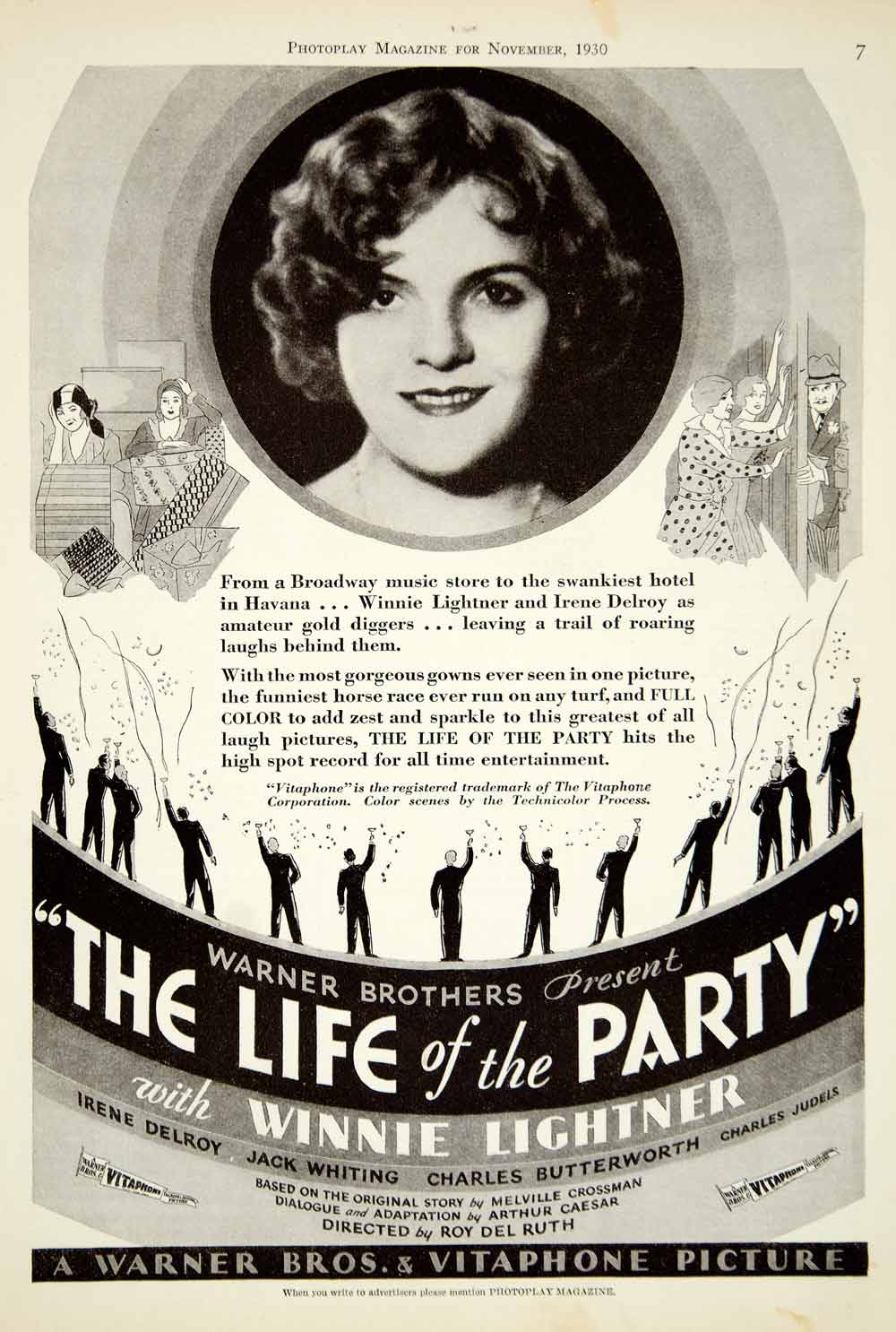This black-and-white movie poster from November 1930, featured in Photo Play Magazine, promotes "The Life of the Party," a Warner Brothers and Vitaphone picture. The top of the poster showcases a circular headshot of a woman with short dark hair and dark eyes. Flanking her image are drawings that hint at scenes from the movie. Central to the poster are two paragraphs describing the film's exuberant plot: Winnie Lightner and Irene Delroy star as amateur gold diggers transitioning from a modest Broadway store to the lavish hotel scene in Havana, leaving a trail of laughter in their wake. The film boasts extravagant gowns, comical horse rides, and vibrant entertainment. Below the descriptive text, a line of men in formal attire hold up glasses in celebration, forming an arc. Beneath this image, the text reads, "Warner Brothers presents The Life of the Party," prominently featuring Winnie Lightner's name, along with additional cast members Irene Delroy, Jack Whiting, Charles Butterworth, and Charles Judales. The poster concludes with, "A Warner Brothers and Vitaphone picture" at the very bottom.